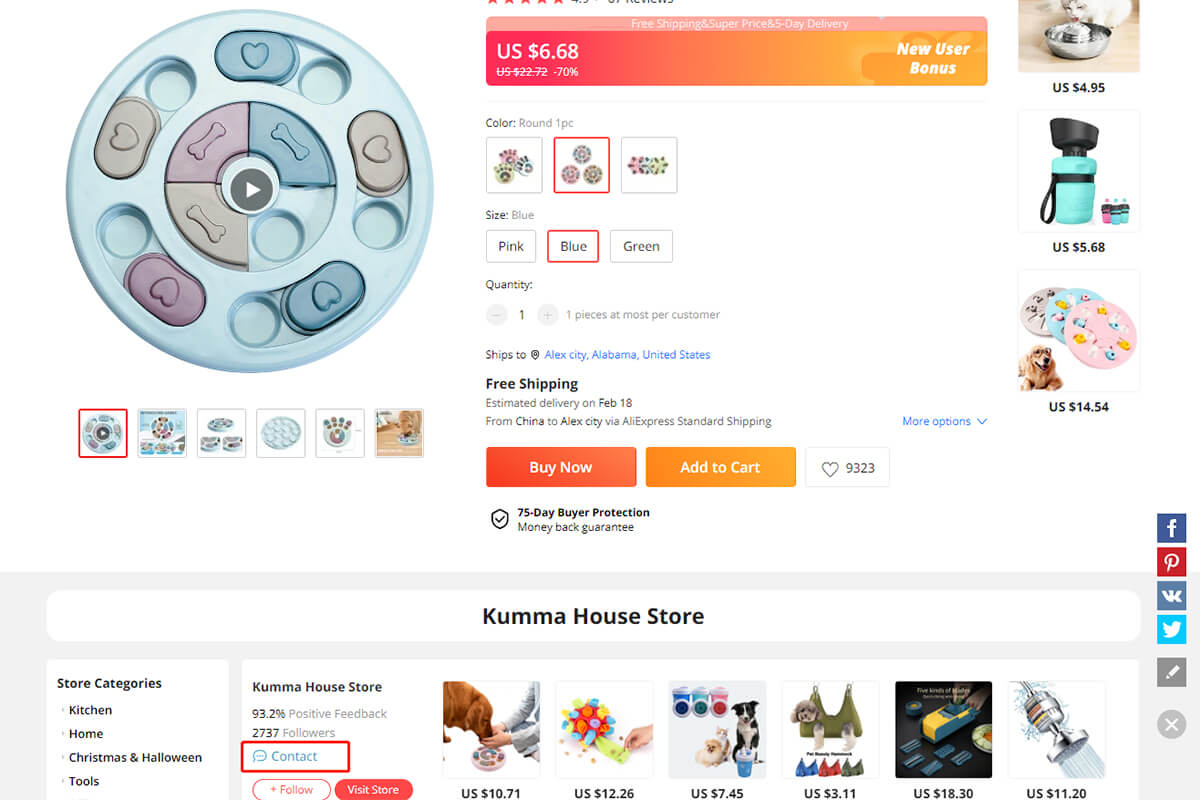The image depicts an online product page for a dog food or treat container designed to engage dogs in a puzzle-like activity to retrieve their food. The item is a circular, teal-colored container adorned with heart and dog bone motifs. Below the main image, there are thumbnail previews of the product from five different angles, allowing the user to click for various views. The price is listed as US $6.68, and there is a mention of a "new user bonus." Options for selecting different colors, sizes, and quantities are also available.

To the right of the product information, there is a section featuring recommended items that might catch the user's interest. At the bottom of the page, the seller is identified as "Kuma House Store," accompanied by a list of store categories, numerical details, and additional product suggestions.